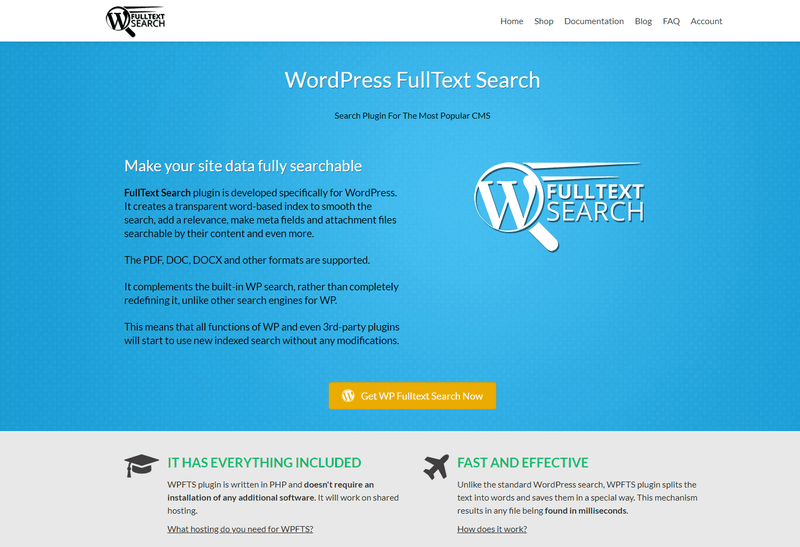The image is a screenshot of a website. At the top left corner, there is a magnifying glass icon followed by the text "Full Text Search." Dominating the center of the page is the heading "WordPress Full Text Search" with a subheading that reads "Search Plugin for the Most Popular CMS." On the left side of the page, a detailed description states: "Make your site data fully searchable. The Full Text Search plugin is developed specifically for WordPress. It targets a transparent word-based index to enhance search relevance. The plugin makes many meta fields and attachment files searchable by their content and supports multiple formats including PDF, DOC, and DOCX. It complements the built-in WordPress search rather than completely redefining it. Unlike other search engines for WordPress, this plugin allows all functions of WordPress and even third-party plugins to utilize the new indexed search without requiring any modifications."